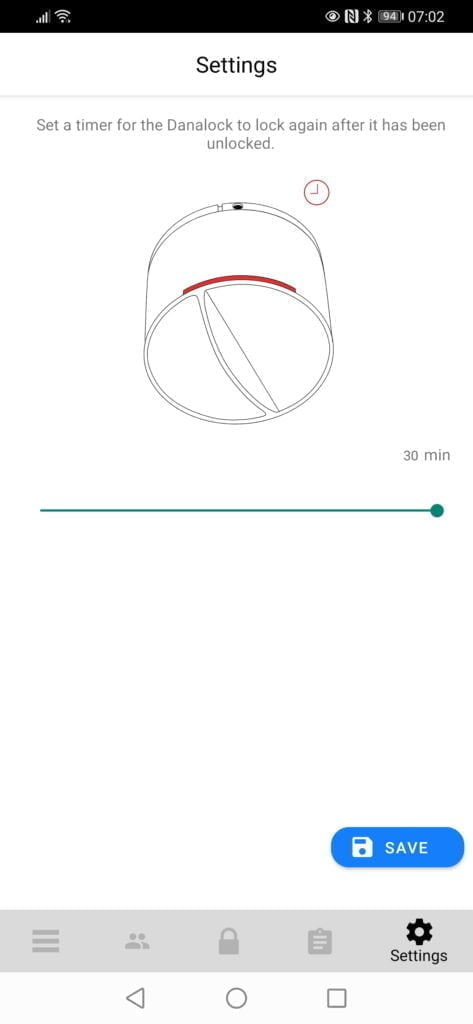This image appears to be a screenshot from a smartphone device. At the top of the image, there is a black status bar displaying Wi-Fi signal strength, battery life, and the current time. Below the status bar, the screen is predominantly white and features the title "Settings."

In the prominent section of the display, there is an important instruction: "Set a timer for the Dana lock to lock again after it has been unlocked." Beneath this text, there is an interface resembling a kitchen timer, complete with a small clock icon above it. A green progress bar underneath the timer indicates a duration of "30 minutes." Additionally, a blue button labeled "Save" is visible near this section.

Further down the screen, several widgets are arranged, including one labeled "Settings" and another that implies functionality to lock or manage contacts. The bottom portion of the screen features typical navigational buttons commonly found on smartphones, such as the back button and other standard options.